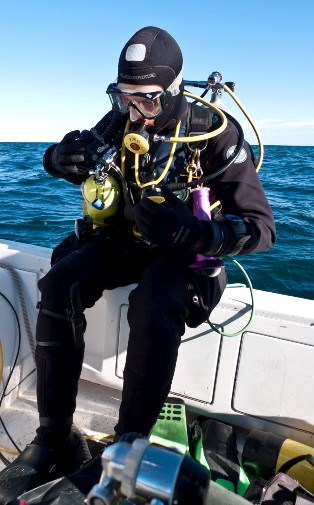The image captures a scuba diver seated on the edge of a white boat, preparing for a dive. He is dressed in full black and white scuba gear, which includes a black hat integrated with his diving suit, goggles, and thick gloves, suggesting he is in a colder region. The diver, turned towards the boat, seems to be inspecting or adjusting his equipment before a backward flip into the ocean. Notably, his gear includes a bright yellow air tank and a slightly duller yellow mouthpiece. A purple object is clutched in his arms, and various colorful items are scattered on the boat's floor, near his feet. The fins still on his feet hint at his imminent dive. The sky above is a clear, light blue with distant clouds, and the ocean behind him glistens in a beautiful grayish-blue hue. A green-like object is positioned next to his left leg, adding another splash of color to the scene.